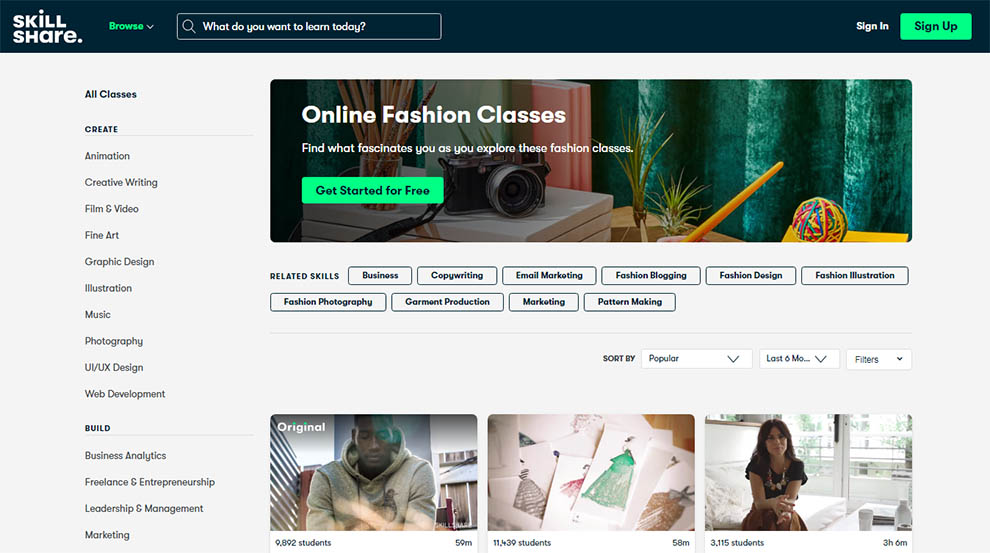This image, taken from the Skillshare website, prominently displays the Skillshare logo in the upper left-hand corner. The logo consists of the word "Skillshare" split into two parts, with "Skill" on top of "Share." The word "Share" concludes with a period. This logo appears within a sleek, black horizontal bar spanning the upper section of the image. 

To the right of the logo, there's a browser icon accompanied by a dropdown arrow, rendered in a light green font. Adjacent to this, a search bar prompts users with the question, "What do you want to learn today?" This search bar is centrally located along the top section. 

On the upper right-hand side, the site features two primary call-to-action buttons: "Sign In" and "Sign Up."

Dominating the central area of the website is a detailed vertical menu situated on the left-hand side. This menu is divided into sections, beginning with "Create," which encompasses various categories such as Animation, Creative Writing, Film and Video, Fine Art, Graphic Design, Illustration, Music, Photography, UI/UX Design, and Web Development. These categories are collectively labeled under "All Classes."

Below the "Create" section, there's a "Build" section, which includes Business Analytics, Freelance and Entrepreneurship, Leadership and Management, and Marketing. 

This comprehensive navigation layout effectively showcases Skillshare's extensive range of learning opportunities, tailored to both creative pursuits and professional development.